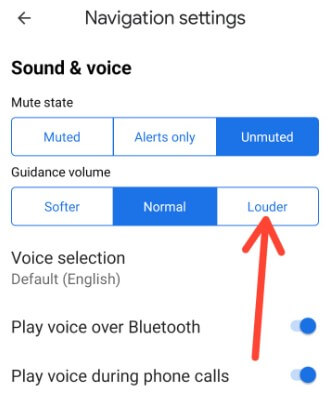The image depicts a screen titled "Navigation Settings" with a back button in the top left corner. The text is predominantly black, with certain elements highlighted in blue. 

On the top left of the screen, there is a section labeled "Sound and Voice". At the bottom, a section labeled "Mute State" is displayed. This section is divided into three horizontally arranged selections: "Mute", "Alert Only", and "Unmuted". These options are outlined in blue and separated by blue lines. "Unmuted" is highlighted in blue with white text, indicating it is the current selection, while "Mute" and "Alert Only" are written in blue on a white background.

The second setting is "Guidance Volume", featuring three options: "Softer", "Normal", and "Louder". The "Normal" option is highlighted in blue, suggesting it is the currently selected volume. A red arrow from the bottom points towards the "Louder" option, indicating the user's next action or a suggestion.

Below "Guidance Volume" is the "Voice Selection" section, with the default set to English. Two settings appear on the left side: "Play Voice Over Bluetooth", which is turned on and indicated by a blue toggle switch on the right, and "Play Voice During Phone Calls", which is also on, denoted by a blue toggle switch on the bottom right.